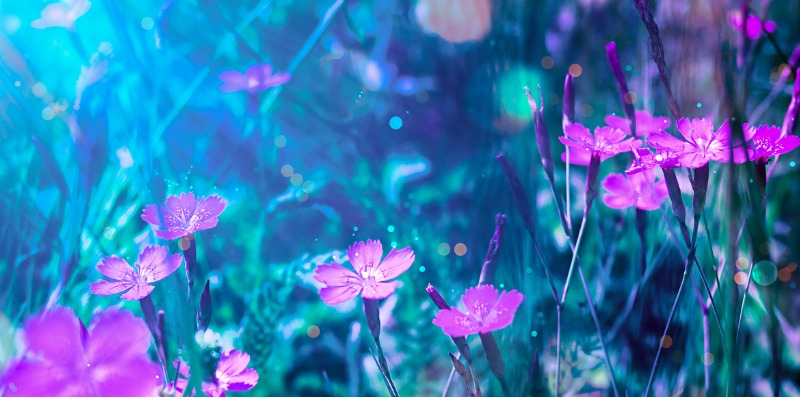This rectangular-shaped photograph captures a serene, nature-inspired scene, possibly taken outdoors during daylight or in a terrarium-like setting. The foreground is dominated by clusters of small, delicate purple flowers, each with five petals. These flowers are affixed to blue or purple stems, which start thick towards the top and thin out toward the bottom. Some flowers are partially bloomed or unbloomed, showcasing purple tips. The centers of these flowers feature hues of white to pink. The background, though blurry, is filled with lush green leaves and multiple stems, suggesting a verdant field. Additionally, the backdrop includes bluish and pinkish dots, resembling orbs where light might be reflecting off various elements. The overall cool-toned palette, with a bluish-purple ambiance and bright light emanating from both sides, gives the image a mystical and almost underwater-like quality.